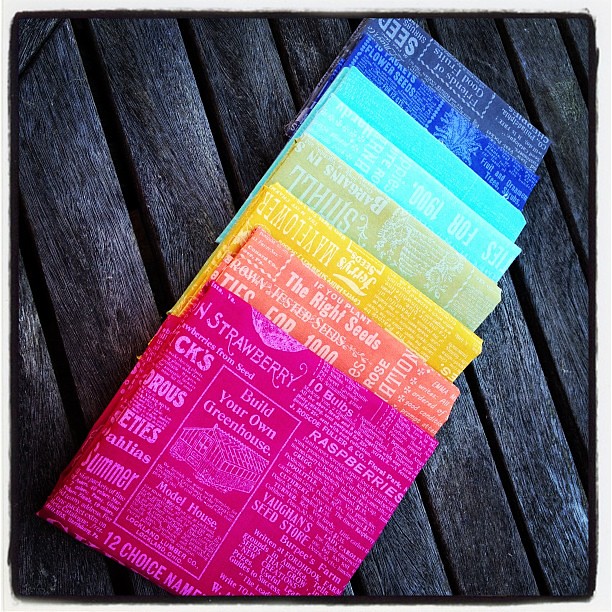This color photograph captures eight vividly colored squares neatly arranged on a background of dark, almost black, painted wooden planks. The squares are stacked in a gradient that mimics a rainbow, starting at the bottom with a very dark blue square, followed by bright blue, vibrant sea green, pale sea green, orange, bright yellow, peach, and finally a vivid pink or fuchsia at the top. Each square appears to be folded, possibly indicating they could be reusable gift bags, bandanas, or different kinds of napkins. The surface of each square is adorned with small, white vintage newsprint text. Detailed inspection reveals the pink square features information about strawberries, building your own greenhouse, and raspberries; the orange one mentions planting seeds and roses; the yellow square talks about May flowers; the sea green one has a picture of a beehive and talks about small bargains; the bright blue piece refers to something from the 1900s; and the dark blue square discusses flower seeds, good fruits, and shrubs. The meticulous overlay of this old newspaper print adds a vintage charm to the vibrant display, creating a visually captivating contrast against the dark wooden backdrop.